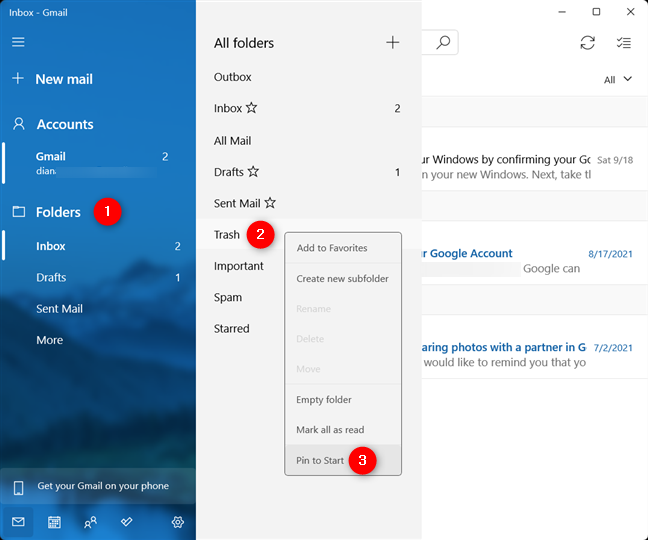This screenshot, likely taken from either a desktop computer or a tablet given its square dimensions, showcases a detailed sequence of actions within the Gmail interface. The image is sectioned into three overlapping areas. 

**Background**: On the right, the main Gmail application displays a classic white background with black and blue text and dated emails from 8-17-2021 and 7-2-2021 visible.

**Left-hand Side**: The far-left column reveals the opened main menu, highlighted in blue, featuring various clickable options. The "Folders" option has a red circle labeled "1" in white, indicating the first step in the process.

**Middle Column**: When "Folders" is selected, the middle column expands to show a list of folder options. The "Trash" folder here is pointed out with a red circle marked "2," indicating the second step in the sequence.

**Foreground Pop-up**: Upon selecting the "Trash" folder, a pop-up appears within this middle column, with the bottom section of this pop-up highlighting the "Pin to Start" option. This option is emphasized with a red circle labeled "3," designating it as the final step in the process.

The careful numbering and highlighting in red circles clearly guide the user through a step-by-step tutorial within the Gmail interface.